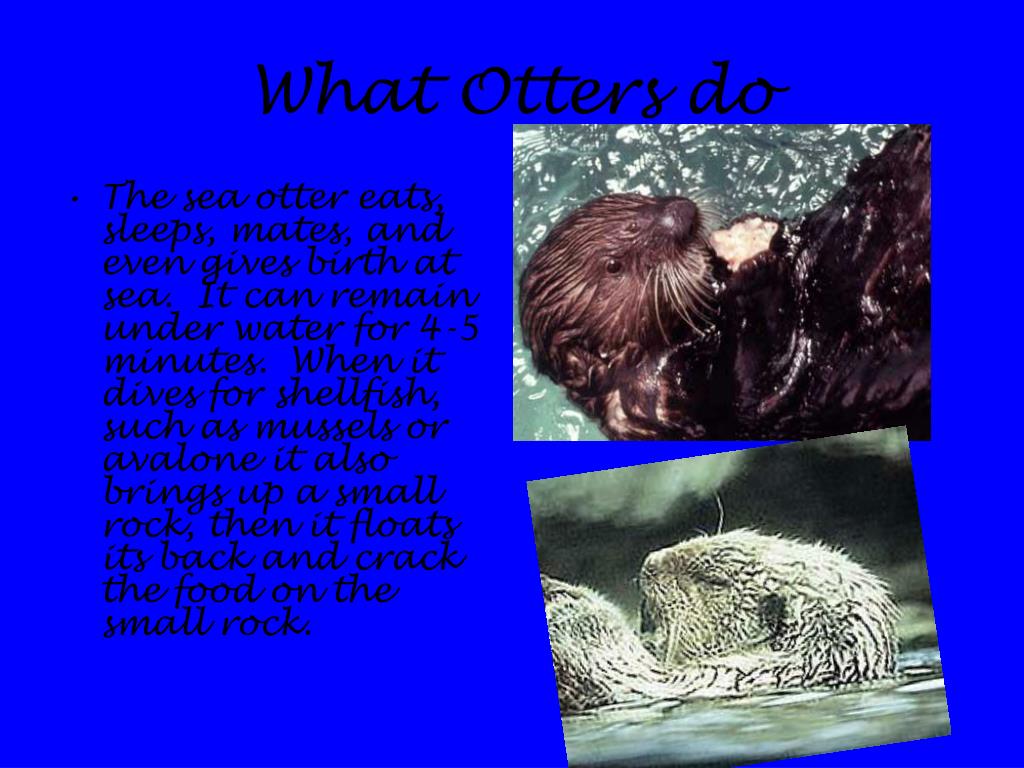The image features a royal blue background with black text in a cursive font. The title at the top center reads, “What Otters Do.” On the right side, there are two photos of otters. The top photo shows a dark brown otter with white whiskers, floating on its back and holding something in its hands, possibly eating. The bottom photo displays a white otter, also with white whiskers, floating on its back with its eyes closed, appearing to be asleep. 

On the left side of the image, a series of informational bullet points describe various behaviors of sea otters. The text explains that sea otters eat, sleep, mate, and even give birth at sea. They can remain underwater for four to five minutes. When they dive for shellfish, such as mussels or abalone, they bring up a small rock and use it to crack open their food while floating on their backs. The background of the top otter's photo includes some white and green specks, adding more context to the scene.